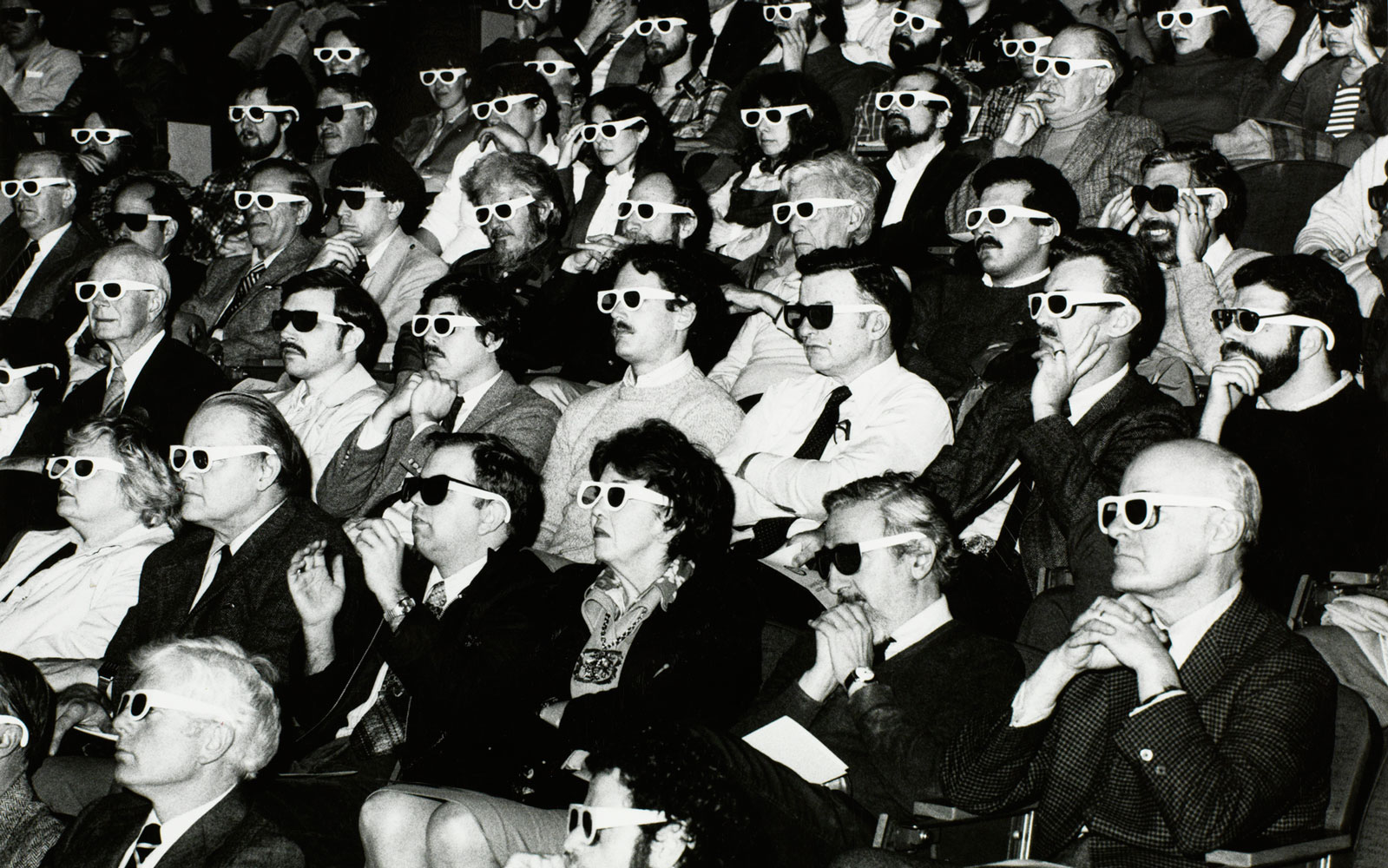This black and white landscape photograph depicts a crowded audience from the 1950s, focusing intently on an unseen film, likely in a movie theater. The audience, consisting primarily of older adults around the age of 40 or 50, is dressed in the formal attire typical of the era, with men in suits, ties, and collared shirts, and women in dresses. Everyone is wearing 3D glasses, which feature distinctive white ear stems, though the frames vary in color, with some being entirely white and others a mix of white and black. A man in the lower left corner, with fluffy white hair, a black suit jacket, a white shirt, and a black tie, stands out for his light skin. Another man, situated to the right, is nearly bald and wears his regular glasses under his 3D glasses, accompanied by a tweed jacket with his hands clasped under his chin. The audience's collective gaze is fixed to the left, deeply immersed in the film they are watching.